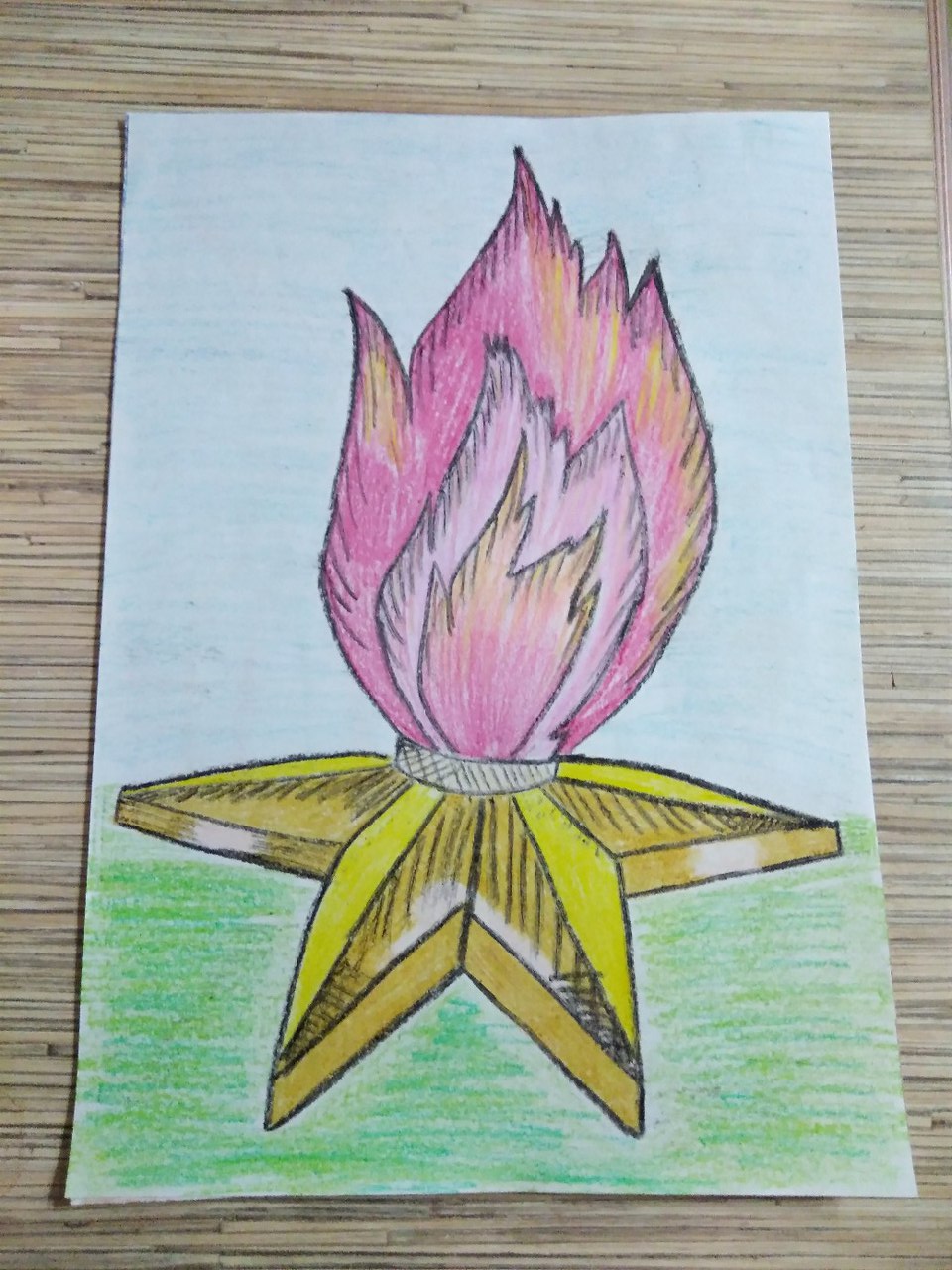This illustration, created using vibrant crayon strokes, is set against a thin, bamboo-like textured surface with a plain piece of paper. The paper appears to consist of two overlapping sheets. The bottom third of the artwork is filled with a rich green hue, while the upper two-thirds showcase a delicate light blue background. Dominating the center of the image is a three-dimensional yellow star, from which vivid pink flames erupt. Encircling the midpoint of this 3D star is a slender ring, acting as the source from which the dynamic flames emanate. The crayon technique infuses the piece with a charming, hand-drawn quality.